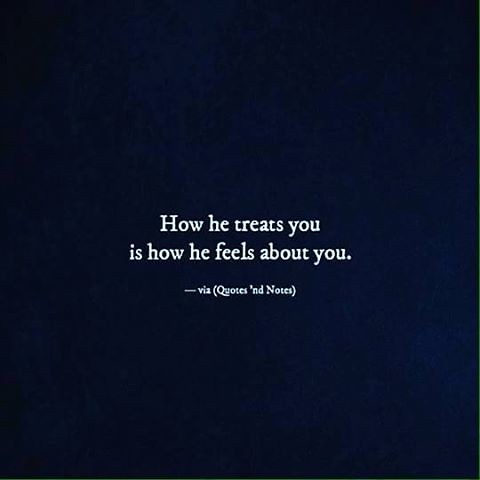This image, suitable for sharing on social media platforms like Facebook or Pinterest, features a square composition with a solid dark blue, nearly black background. Positioned in the center is a plain white font delivering a quoted message. The text reads: "How he treats you is how he feels about you." Below this, a smaller line indicates the source, marked with a dash followed by "via 'quotes' and 'notes'" within parentheses. The minimalistic design and profound message make it a shareable piece of digital content.